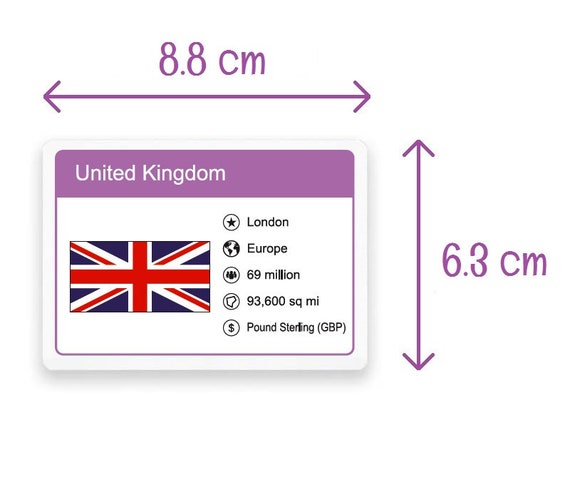The image depicts a rectangular information card about the United Kingdom, approximately the size of a credit card, with dimensions specified as 8.8 cm in width and 6.3 cm in height. This measurement detail is illustrated with purple arrows pointing left and right for the width, and up and down for the height, positioned beside the card. The card itself has a prominent purple banner across the top, stating "United Kingdom" in white text. Below this banner, the card's background shifts to white and contains various informative graphics and text. 

On the right-hand side, there's a star symbol accompanied by the text "London." Next to it is an illustration of a globe labeled "Europe." Further down, the population is denoted as "69 million," followed by the area "93,600 square miles." At the bottom of the card, a dollar sign encircled indicates the currency as "Pound Sterling (GBP)." Additionally, there is a depiction of the United Kingdom's map colored in blue, white, and red. The overall design features a purple border, thicker at the top compared to the sides and bottom.